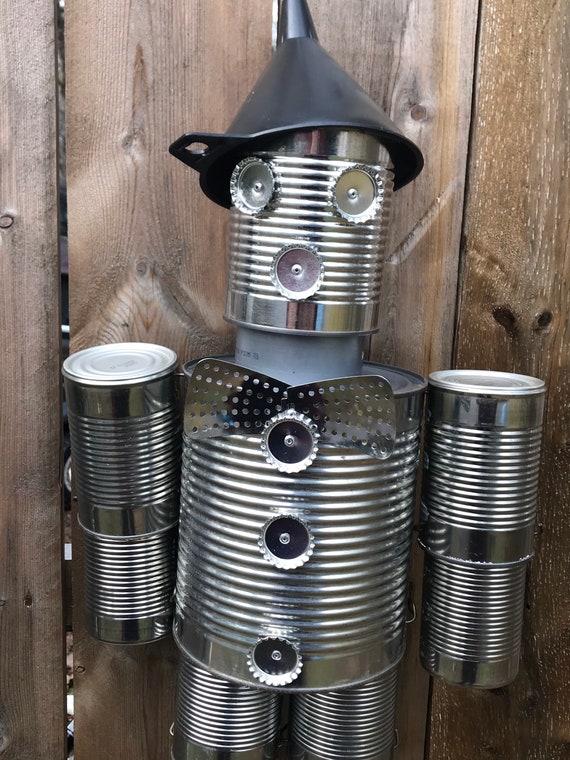A captivating piece of artwork depicts a whimsical robotic creature, characterized by its inventive use of everyday objects. The robot's head is adorned with a black oil spout serving as a hat, giving it a vintage touch. The face is creatively assembled using three bottle caps, which add quirky facial features. Its body is constructed from a can, complete with three bottle caps positioned as buttons down the torso. Adding a touch of formality, the robot sports a bow tie and holds a spatula, hinting at a playful personality. The arms are ingeniously made from two additional cans, while its legs are also formed from cans, providing a sturdy and cohesive appearance. The entire scene is set against the rustic backdrop of a wooden fence, highlighting the contrast between the mechanical whimsy of the robot and the natural texture of the wood.